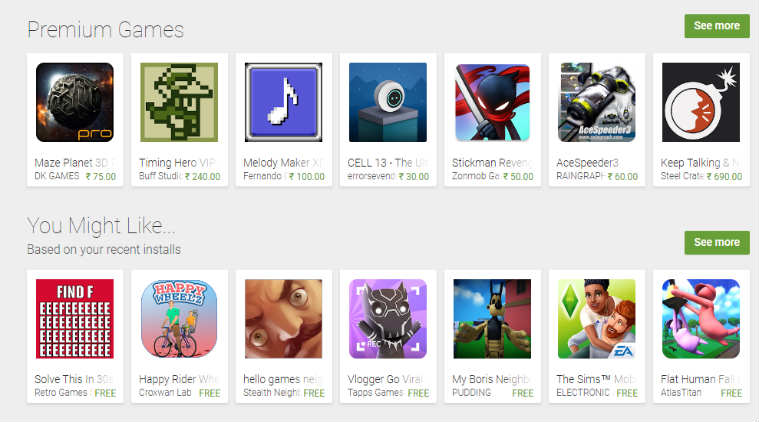This image captures the interface of an Android app store, characterized by its distinct green and light gray color scheme. There are two primary sections visible, each showcasing different categories of games.

At the top is the "Premium Games" section, containing a curated list of seven titles:
1. Maze Planet
2. Timing Hero VIP
3. Melody Maker
4. CELL 13
5. Stickman
6. Ace Speeder 3
7. Keep Talking

Below this is the "You Might Like" section, which suggests games based on recent installs. The titles in this list include:
1. Solve This in Three
2. Happy Writer
3. Hello Games
4. Water Go Viral
5. My Boris Neighbor
6. The Sims
7. Flat Human

Next to the title of each game, the name of the publisher is visible, along with the price, which can be either in a specific currency or listed as free. Notably, all games in the "You Might Like" section are free, whereas the "Premium Games" are paid.

Each section has a "See More" button positioned to its right, allowing users to explore additional games beyond the initially displayed titles.